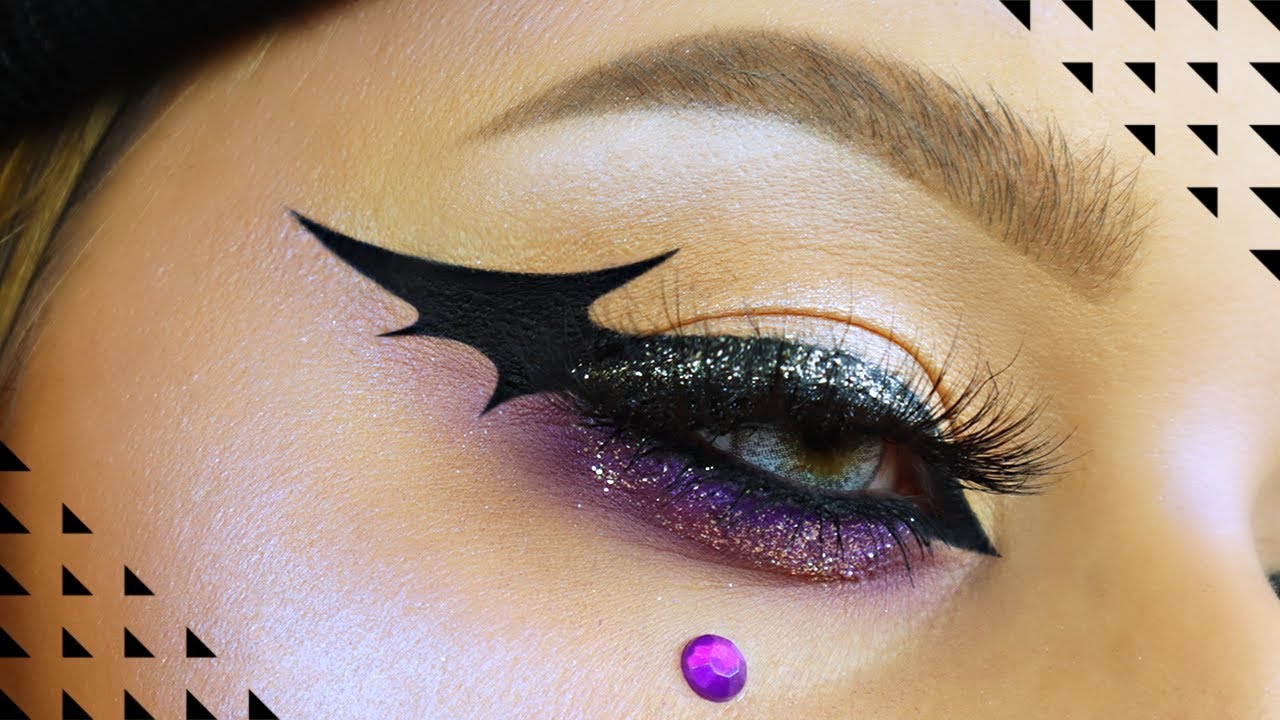In this AI-generated image, we see a close-up of the right side of a person's face, focusing on an intricately made-up eye. The person's blue eye, featuring a hazel center, appears half-closed. Their well-shaped, filled-in brow arches perfectly, accented by the spiked-up brow powder. The eye makeup is a striking bat wing design, created with black eyeliner that extends dramatically from both the top and bottom lash lines. The upper lid lacks eyeshadow, while the bottom lash line is adorned with purple glitter liner, adding a sparkling contrast. Small black triangles are strategically placed on the cheek and in the upper right corner of the image, drawing attention. Additionally, a tiny purple jewel embellishes the area just beneath the eye. The person's skin has a glossy sheen, emphasizing the crisp details of the elaborate makeup. The entire composition is framed to showcase the eye, eyebrow, a hint of the nose, and part of the cheek, with an overall aesthetic resembling a makeup advertisement.